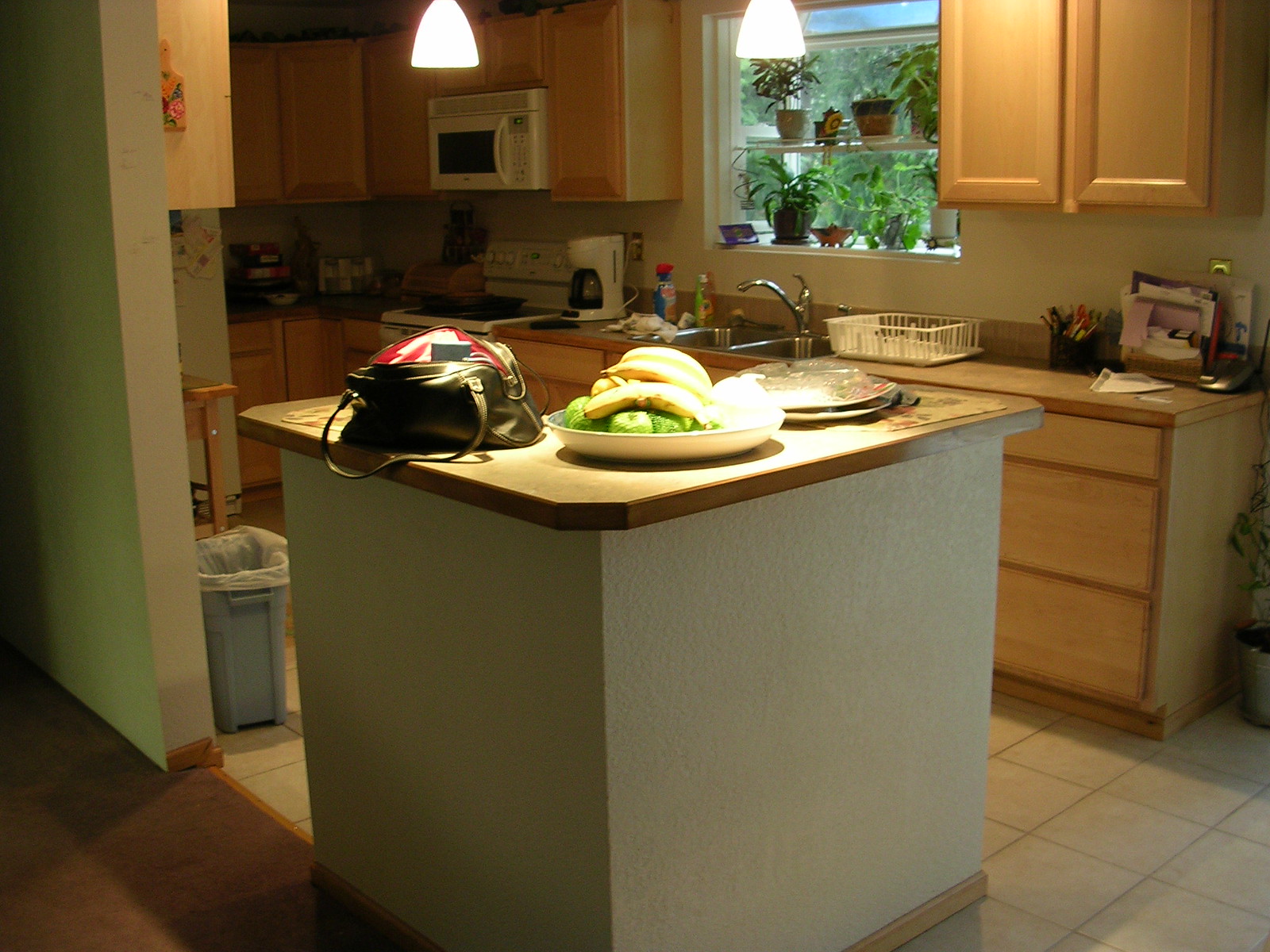This candid photograph captures a cozy, J-shaped kitchen with a slightly dim lighting that gives it a lived-in ambiance. Central to the scene is a unique, bar-height kitchen island that appears to be either square or triangular. It features white paneled sides and a light wood countertop, reminiscent of a butcher's block.

In the background, the kitchen cabinets are made of the same light-colored wood, harmonizing with the warm, natural tones of the island. The countertops of these cabinets are similarly light, possibly pink or another shade of butcher's block wood, creating a cohesive aesthetic throughout the kitchen. The cabinets line most of the back wall and seamlessly extend into the side wall, contributing to the kitchen's J-shaped layout.

The white walls provide a clean backdrop, while tan ceramic tiles cover the floor, adding a touch of rustic charm. A glimpse of a hardwood floor appears in the bottom left of the image, hinting at the adjoining space. 

A window placed centrally at the top of the photograph allows natural light to filter into the room, although the foliage outside suggests a shaded view. The windowsill serves as a space for a few potted plants, adding a refreshing touch of greenery to the kitchen. A small shelf above the window further personalizes the space, enhancing its homey feel.